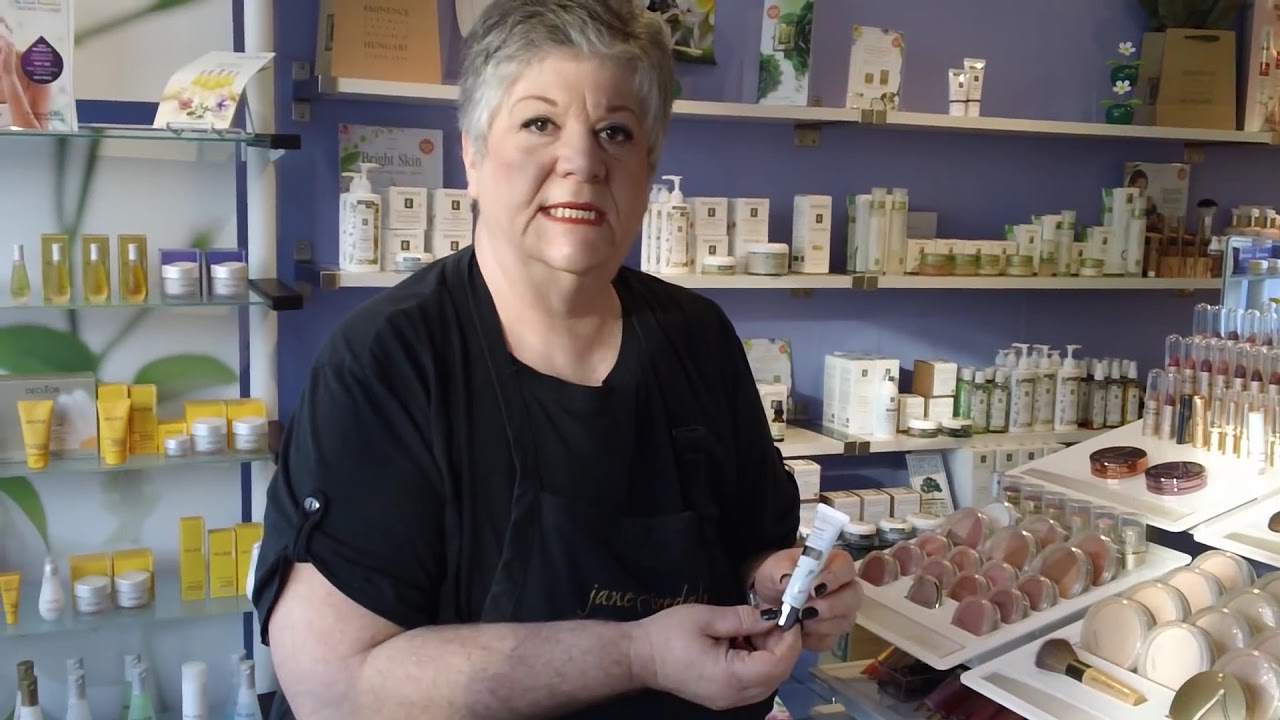In this rectangular image, an older woman, likely in her 70s, stands almost centered within a beauty supply store. She has short, cropped gray hair and is slightly overweight. Her attire consists of a black short-sleeved top and possibly a black apron with a business logo. She wears red lipstick and her fingernails are painted with dark lacquer. The woman holds a white tube of a skincare or makeup product with a silver cap and some gray markings, possibly lotion, in front of her as she looks directly at the camera.

Behind her, a blue wall adorned with horizontal shelves is visible, displaying various cosmetic items in rectangular boxes, primarily white with dark gray or black writing, and other assorted containers. To her right, the shelf continues along a white wall with green leaf patterns, stocked with an array of yellow and white products in tubes and boxes. In the lower right-hand corner, a cosmetics counter can be seen, showcasing round containers of both pink and white makeup, likely powders and blushes. Further to this side is a makeup display featuring eyeshadows, blushes, and lipsticks, enhancing the vibrant and bustling ambiance of the store.